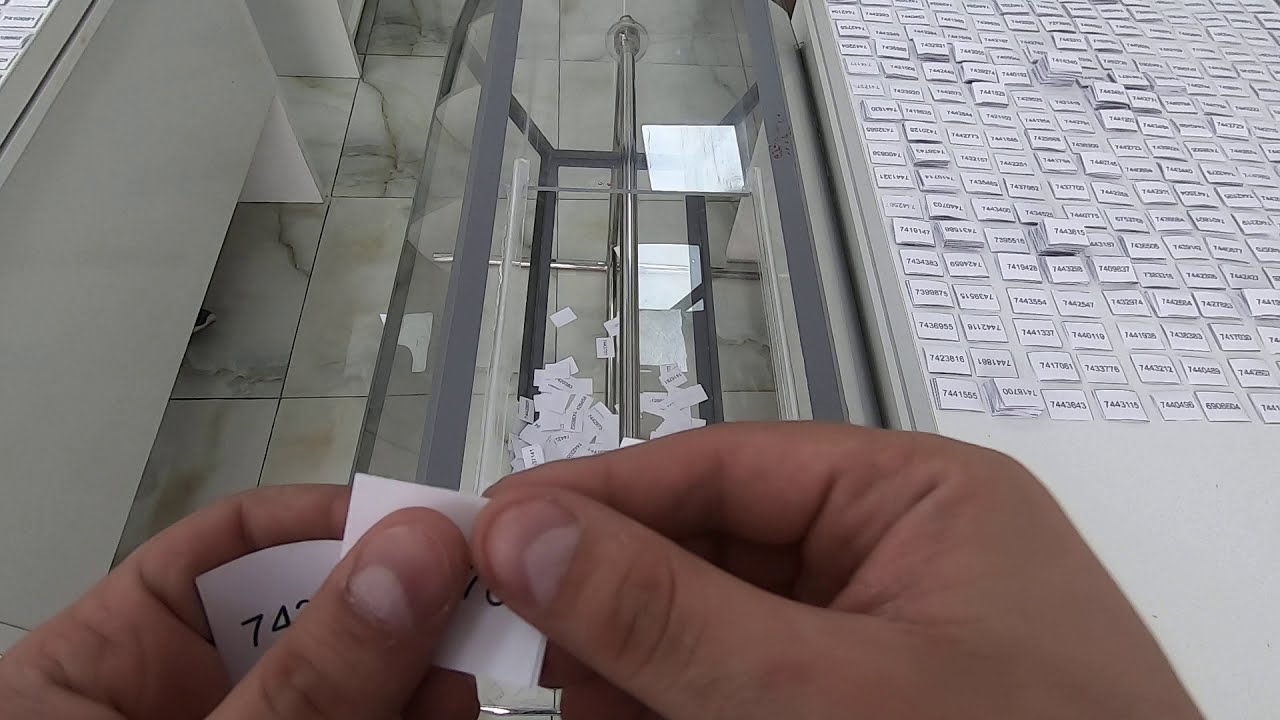A person is captured in the act of holding and throwing two square pieces of white paper, each inscribed with numbers beginning with 7, into an open-door pentagonal spinning device. This device, featuring see-through acrylic sides supported by a gray frame and a prominent silver rod running through its center, already contains multiple numbered squares. The man’s front paper reads "7," while the back one displays "74." To the right, neatly organized stacks of similar white squares—most numbers starting with 7—occupy a table. The scene unfolds atop a white and gray marble tile floor, as the person engages with the device, perhaps sorting or organizing the numbered papers.